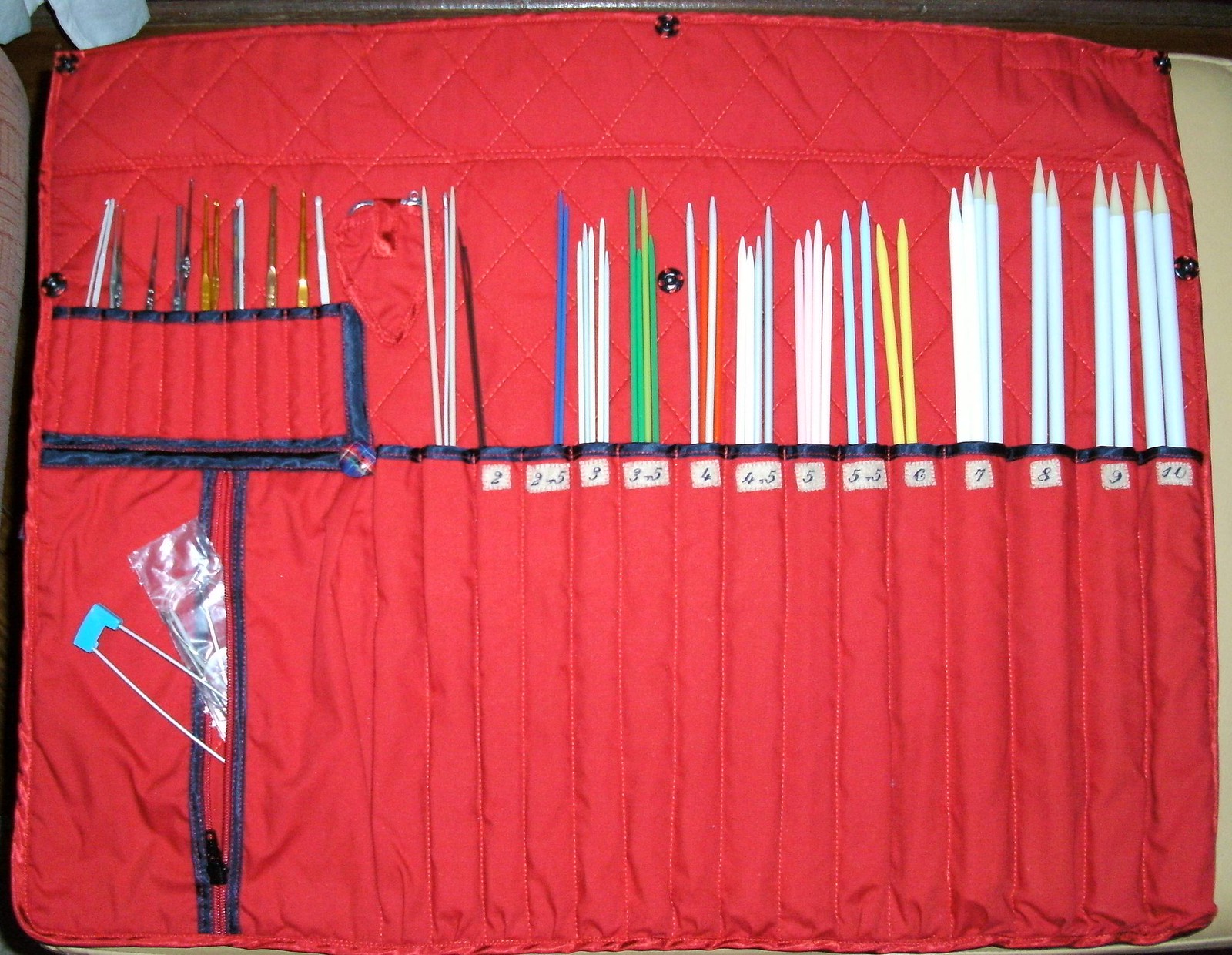This image showcases a detailed close-up of a handmade, quilted red fabric organizer designed for knitting and crochet tools. The organizer, which appears to unroll for use, features a series of stitched sections and narrow pockets, each labeled with black numbers on white fabric, indicating the sizes of the netting needles or knitting needles it holds. These needles are mostly white, with some green ones in the middle and yellow pairs towards the right. They are arranged with the larger ones towards the right and the smaller ones towards the left.

The left-hand side of the organizer includes shorter pockets, housing a variety of crochet hooks and other sewing tools. Notably, there's a pocket bordered in navy blue containing various sewing tools or needles. At the bottom of the organizer, there is a zipper pouch, from which a couple of safety pins—one with a baby blue tip and another still wrapped in plastic—are protruding. Overall, the organizer meticulously stores a vast array of knitting and crochet tools, neatly arranged and easily accessible.